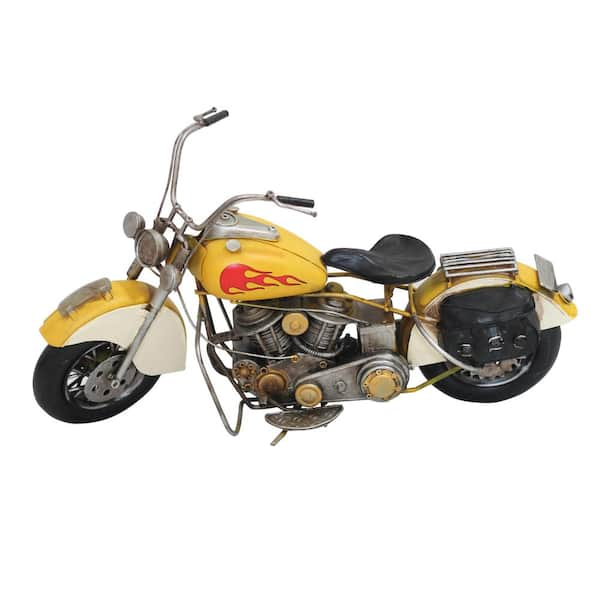This image features an antique-style motorcycle set against a white background. The motorcycle is predominantly mustard yellow, with the front and rear fenders showcasing white panels on their sides. The yellow fuel tank is adorned with a striking red flame design, adding a vivid contrast. Both the front and rear fenders, as well as the tank, are in this mustard yellow shade, combining with the white panels for a classic look.

The bike is equipped with black leather accessories, including a saddle seat and a leather saddlebag positioned against the back wheel. The engine has a steel appearance, accented with gold-painted caps on some components, while the handlebars are basic with black rubber grips.

Additional features include a metal grid rack located behind the seat, suitable for bungee cords or other storage needs. The motorcycle has short, fat wheels and wider handlebars with visible silver brake cords. The bike's overall condition appears to be aged and somewhat worn, with signs of rust indicating it needs maintenance to be fully operational. The image highlights the vintage allure and the well-loved character of this classic motorcycle.